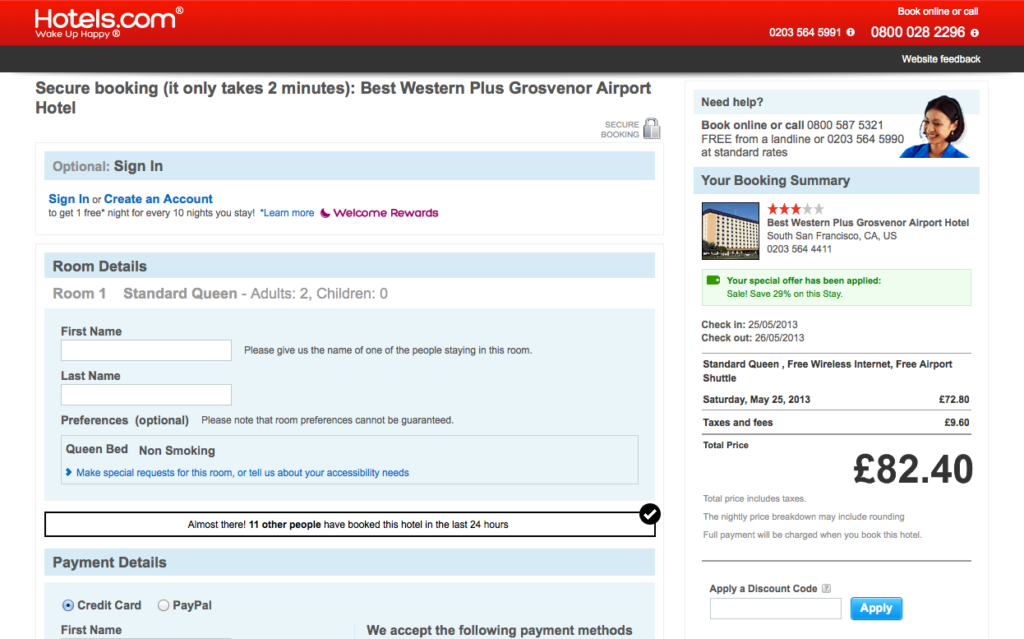The image appears to be a screenshot of a Hotels.com booking page on someone's computer. The interface features a red border at the top, and in white text on the upper left corner, it displays "Hotels.com." On the upper right, there is an option to "Book Online or Call," accompanied by an 800 number. In the center, a message assures users of a "Secure Booking" process that "only takes two minutes."

The screenshot details a reservation for the "Best Western Plus Grosvenor Airport Hotel." Beneath this, there is a section prompting users to "Sign In or Create an Account." Below this prompt, blue text labels a section for "Room Details," specifying "Room 1: Standard Queen, 2 Adults, 0 Children." There are input boxes labeled "First Name" and "Last Name," and it is noted that the person has selected a "Queen, Non-Smoking" room.

Further down, the "Payment Details" section indicates that the user has chosen to pay by credit card. On the right side of the image, alongside a visual of a female figure, there is a "Need Help?" section. Also present on the right is a "Your Booking Summary" in blue text, reiterating the "Best Western" booking with orange three-star rating icons beside it. A green box highlights that a "special offer has been applied," bringing the total price to $82.40.